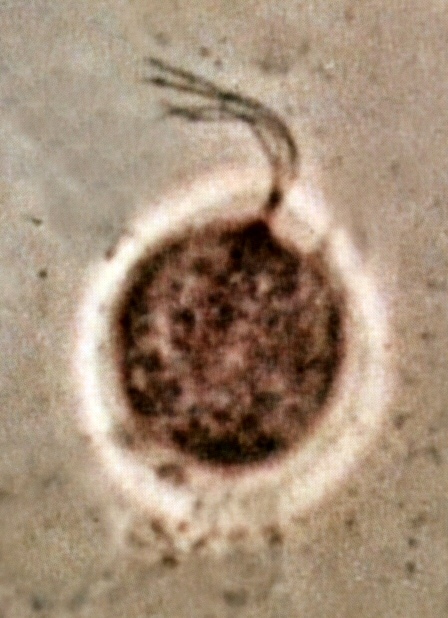The image appears to be a low-resolution, blurry microscopic image showcasing a round, brown blemish on what seems to be human skin. This central entity, potentially a microbe, is distinguished by its tan and black coloration, with several tentacle-like structures extending from its form. Encircled by a white ring, the blemish faces downward in the middle of the frame, set against a dark, soupy background. The overall scientific setting of the image lacks any text, accentuating the detailed, yet somewhat unclear visual elements that give it a rather dirty and brownish appearance.